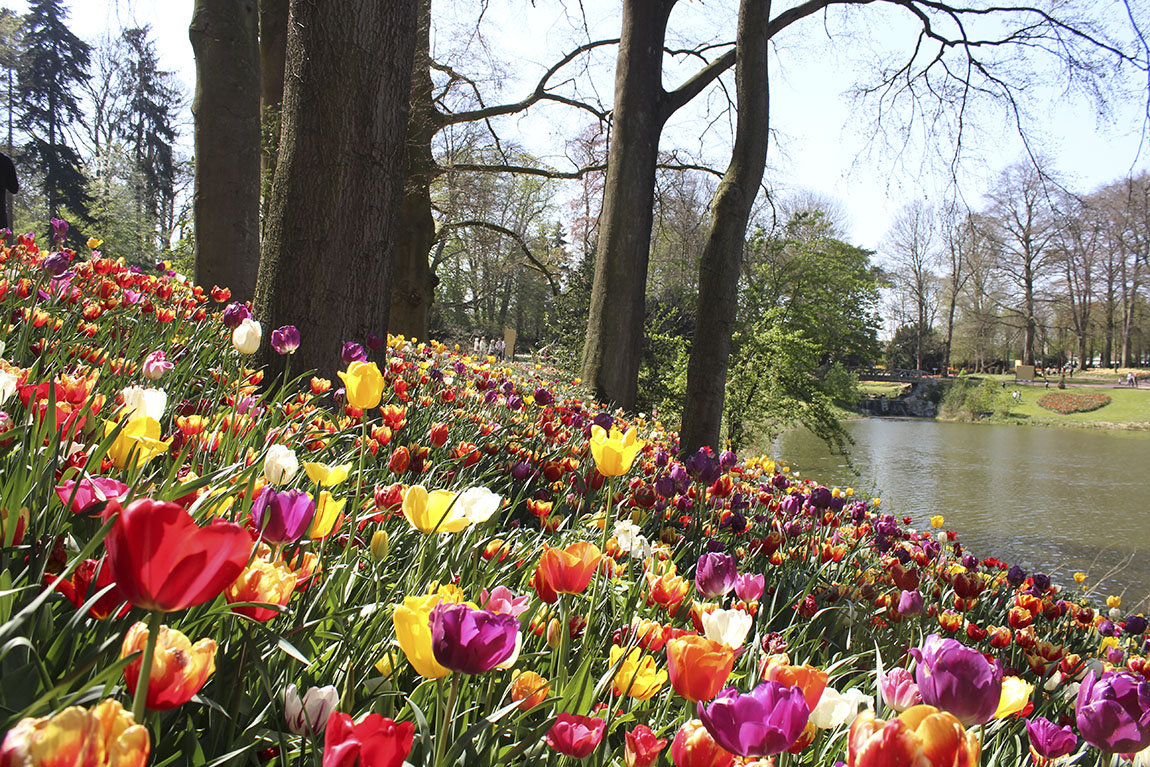In this vibrant photo captured on a bright sunny day, we see a picturesque park scene dominated by a hillside lushly adorned with a myriad of tulips in vivid hues of red, yellow, white, and purple. The hill, enveloped in these colorful blossoms, stretches down towards a body of water that seems to be a lake or a man-made stream, its banks lined with majestic trees. In the distance, the water is crossed by a bridge, adding a quaint charm to the landscape. The park is alive with activity; tiny figures of people can be seen wandering along the trails, some enjoying the playground equipment farther off. A heart-shaped flower bed adds a unique touch to the scene, hinting at careful landscaping. The day, marked by clear blue skies, highlights the seasonal beauty with trees either just budding or stripped of their leaves, suggesting spring or fall. Overall, this serene snapshot captures a vibrant assortment of tulips, the play of light and shadow on the greenery, and the gentle hum of daily park life.